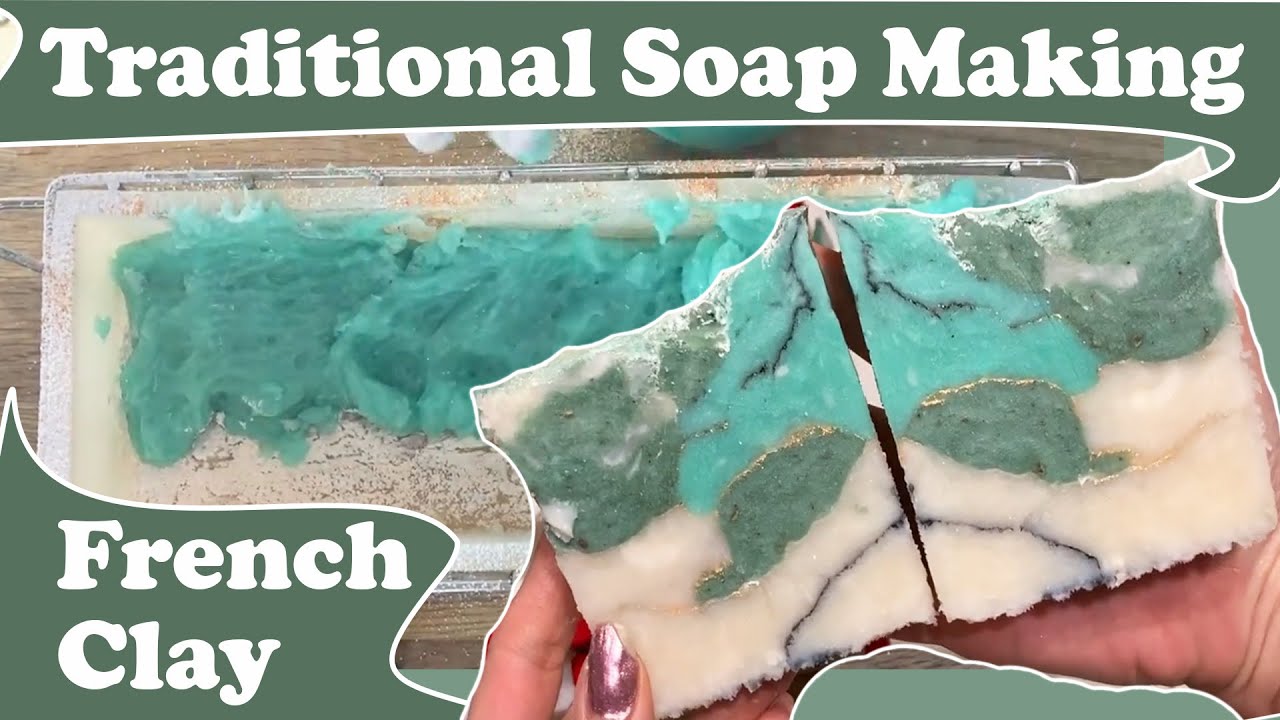The image is an advertisement for traditional French clay soap making, set against a sea foam green background with white text that reads "Traditional Soap Making" across the top. Prominently featured is a white, creamy block of soap with intricate marbling in shades of gold, turquoise, teal, and black. Captured from a bird's eye view, the image showcases the soap before it is cut. Superimposed in the foreground is a close-up of hands with glittery pink, mauve-colored nail polish, holding two cut pieces of the soap, highlighting its layered and marbled texture. The lower left corner of the image displays the text "French Clay" in white against the sage green backdrop, reinforcing the artisanal and traditional aspect of the soap making process.